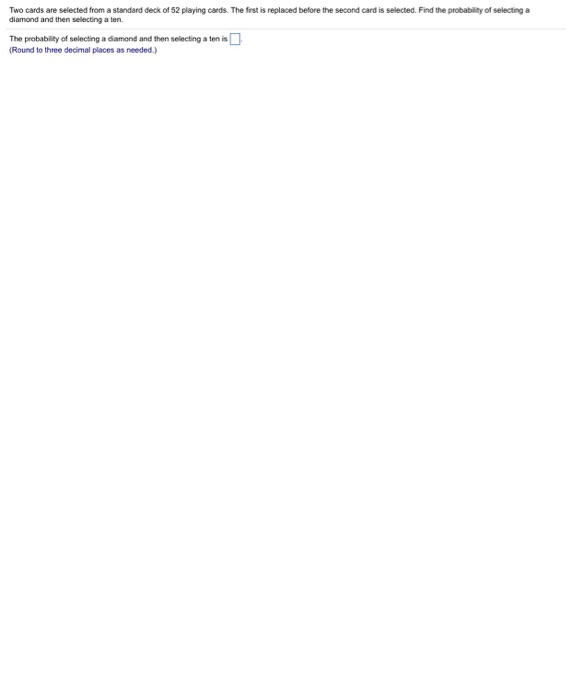The image displays a math problem on a mostly blank page. At the top, there is a prompt in small text that reads: "Two cards are selected from a standard deck of 52. The first is replaced before the second card is selected. Find the probability of selecting a diamond and then selecting a 10." Below this prompt, there is a space to fill in the answer, followed by instructions: "The probability of selecting a diamond and then selecting a 10 is (round to three decimal places as needed)." The task essentially asks for the probability calculation involving selecting cards with replacement. The correct probability involves multiplying the probability of drawing a diamond (13/52) by the probability of then drawing any 10 (4/52), resulting in the combined probability.